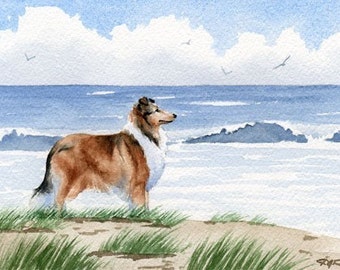The image is a detailed watercolor painting of a serene beach scene featuring a beautiful collie dog. The dog stands majestically on a sand dune covered with green seagrass, gazing thoughtfully towards the right. Its fur is a striking blend of auburn, reddish blonde, and black on its tail, complemented by a furry white chest and a reddish-blond face.

In the background, a tranquil sea stretches out under a vivid blue sky, where puffy white clouds float gently and seagulls soar above the ocean. Small waves crash against the rocks near the shore, creating foamy splashes. The overall composition, rich in texture and detail, evokes a sense of tranquility and the dog's longing to explore the shimmering waters.